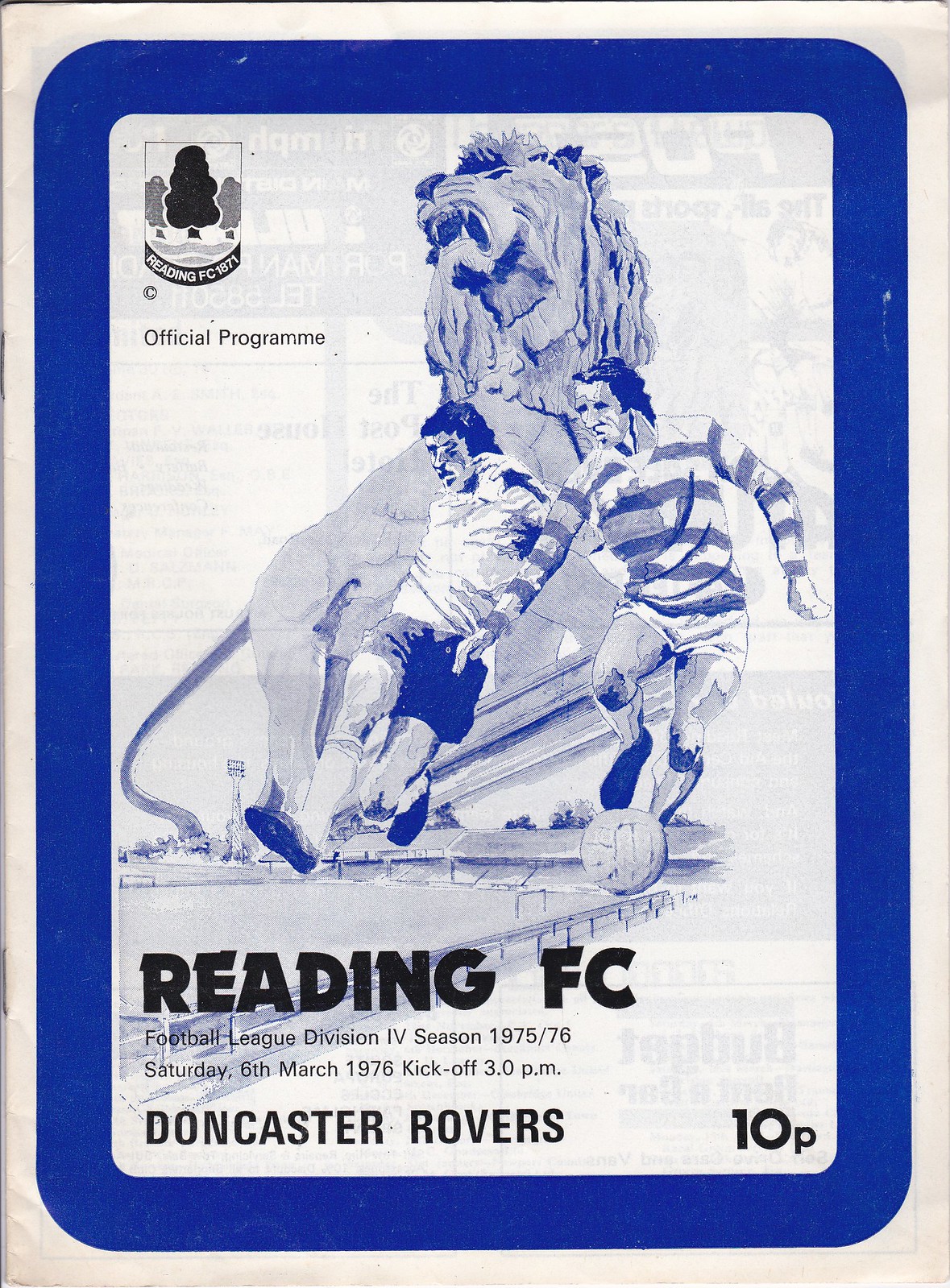The image is a depiction of a faded, weathered official program for Reading FC. The program is printed on thin, white paper, revealing some of the text from the opposite side. It features a thick blue rectangular border reminiscent of a baseball card. In the upper right corner, there is an icon of trees with the text "Reading FC 1871 Official Program." At the center, there's a striking blue sketch of a roaring lion on a rock, with two soccer players depicted in front – one wearing a white shirt with blue shorts, and the other in a white and blue long-sleeve shirt with white shorts – both vying for a soccer ball. Below the central imagery, in bold black font, it reads "Reading FC," followed by "Football League Division Four Season 1975-76," "Saturday 6th March 1976," "Kickoff 3 p.m." The lower right corner indicates the opposing team, "Doncaster Rovers," with a note of the price, "10p." There is also a sketch of a large soccer field in the lower left corner, adding further detail to the cover.